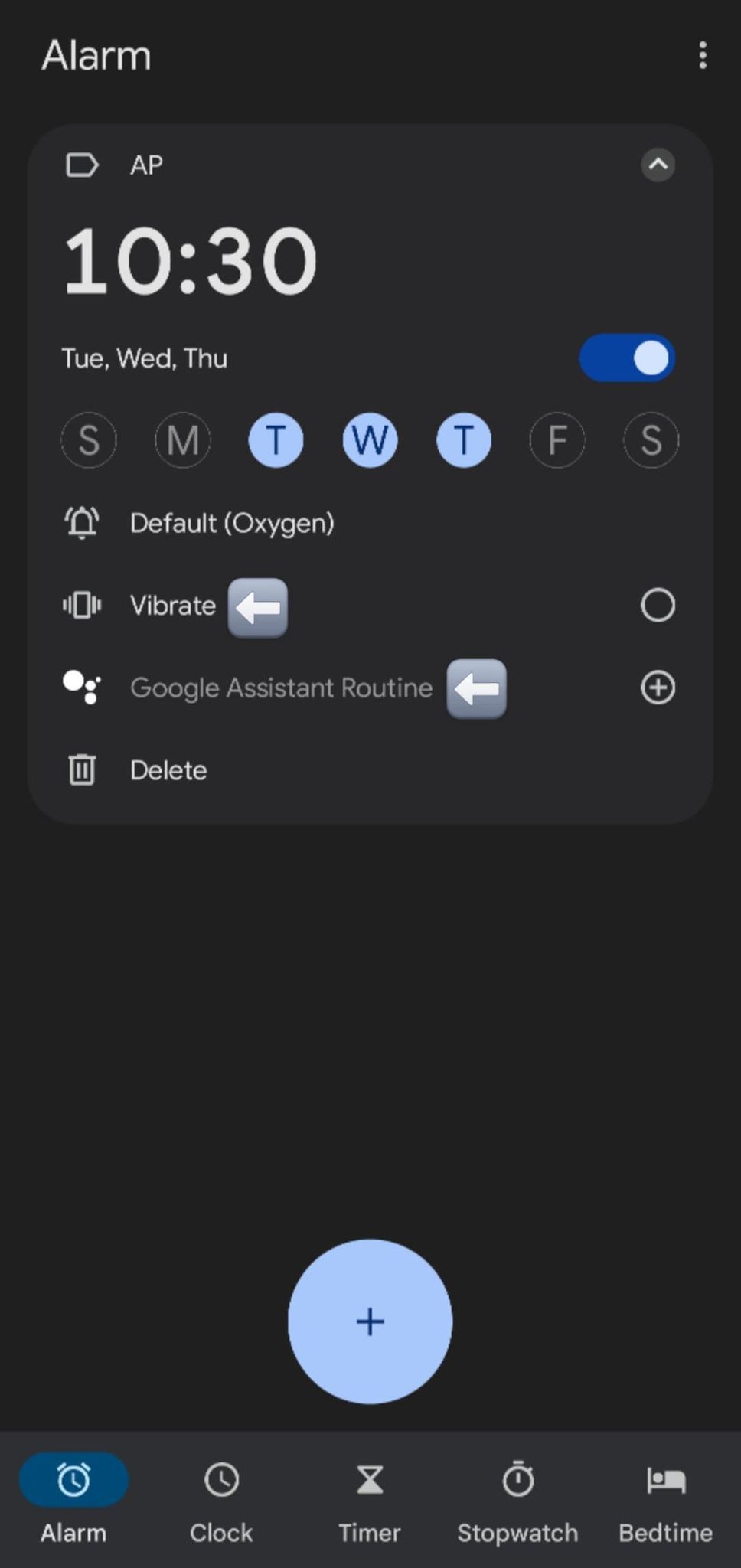This image is a screenshot displaying the alarm settings page of a smartphone, featuring a black background and a light grayish-black overlay box. At the top of this overlay, the word "Alarm" is clearly written in white on the left-hand side, while on the right-hand side, there are three vertical dots indicating a menu option. Within the darker gray portion of the overlay, detailed alarm information is provided.

The alarm is set for 10:30 AM and is scheduled to go off on Tuesday, Wednesday, and Thursday. The days of the week are represented by initials (S, M, T, W, T, F, S) shown in circles with Tuesday, Wednesday, and Thursday highlighted in a lighter blue color, indicating they are selected. There is an active toggle switch next to these days, confirming the alarm is enabled.

Below this section, the ringtone is listed as "Oxygen," the default alarm tone. Additionally, there is a toggle switch with an arrow for the "Vibrate" option and another arrow pointing to the "Google Assistant Routine" feature. Further down is a trash icon labeled "Delete," offering the option to remove this alarm setting.

At the bottom of the screen, a larger light blue button with a blue cross in its center allows for adding new alarms. The bottom menu bar features icons and labels for various functions: Alarm, Clock, Timer, Stopwatch, and Bedtime.